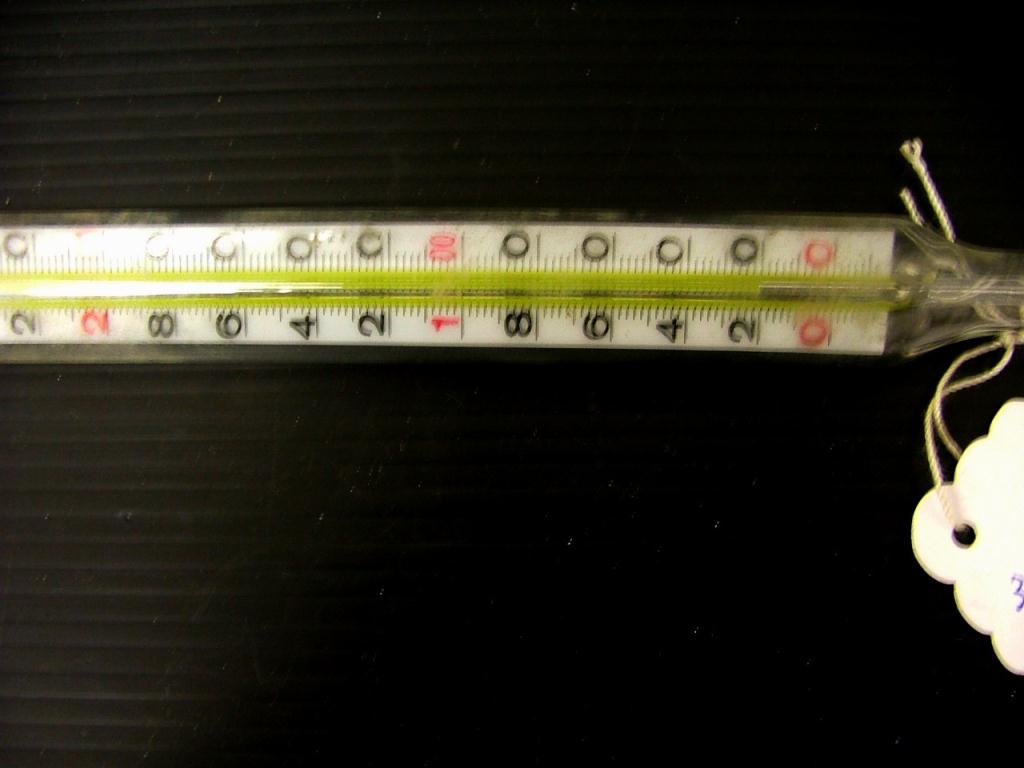A horizontally oriented thermometer is depicted, with the view angled from the bottom-left towards the top-right. The thermometer features a series of numerical markings starting at 0 at the bottom and incrementing by 20 units up to 100, continuing again at intervals from 120 to 200. The center of the thermometer showcases a liquid column, presumably mercury, encased within a metallic strip. Surrounding the metallic strip, the thermometer has a yellow casing. Dash lines are present between the 40-degree intervals for finer measurement reading.

The device is slightly tilted to the left, with a rope tag hanging on its right side. This tag is attached to a small white emblem, which is pinned onto the thermometer. Additionally, a brief storyline or inscription is drawn on this tag. The entire setup is mounted against a black background that has a textured pattern with stripes and slight bumps, providing contrast to highlight the features of the thermometer.